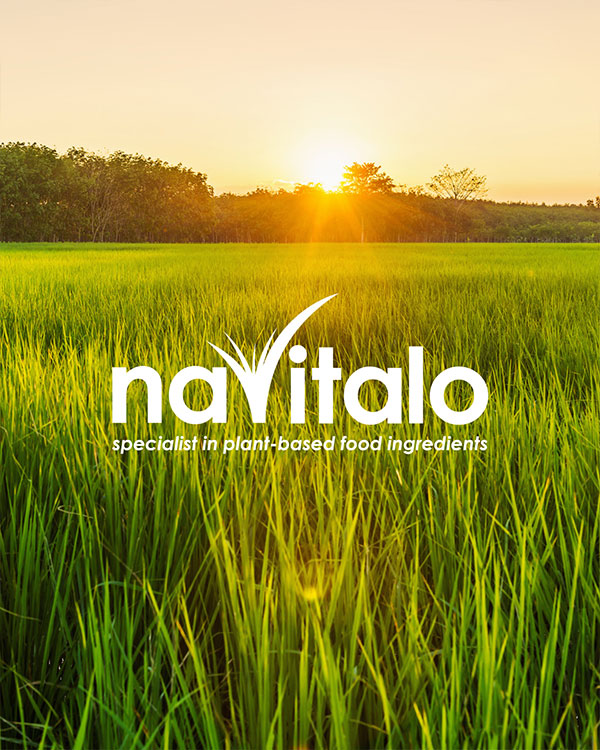This advertisement features a rectangular photograph, approximately six inches high and four inches wide, taken outdoors during either the evening or early morning hours. The image prominently displays a sprawling field of tall, thin grass occupying the bottom two-thirds of the frame. A bold white text in the center reads "Navitalo," with a unique "V" stylized as the top of a plant with little spikes. Beneath this in smaller white print is the tagline, "Specialist in Plant-Based Food Ingredients." The upper portion of the image showcases a row of green trees along the horizon, above which a bright white sun illuminates the sky with hues of peach and golden light. This radiant sunlight casts yellow and orange glows onto the grass below, enhancing the natural beauty of the landscape. The serene and vibrant setting suggests a sunrise, with the sun's rays highlighting the field, trees, and sky, creating a harmonious and inviting scene ideal for an advertisement.